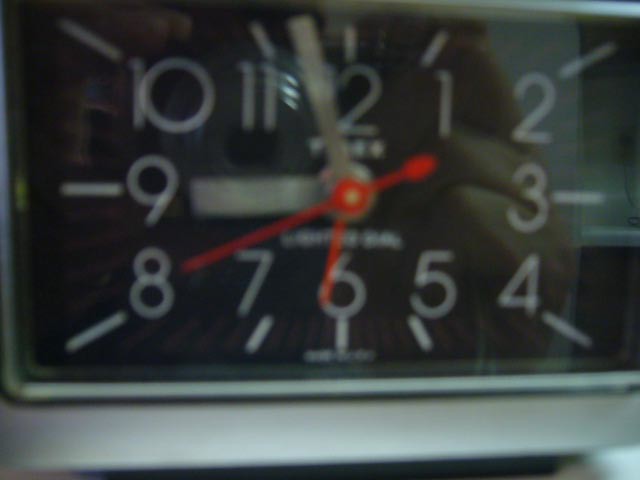An up-close, slightly blurry photograph of a rectangular-shaped clock with a sleek silver bottom. The clock's background is black, adorned with white numerals and notches. The hour and minute hands are silver, while the second hand stands out in red. The time displayed is 8:48, with the second hand positioned over the number 8. The image captures a reflection of the photographer's hand and their silver camera, likely contributing to the blur from potential motion or focus issues.